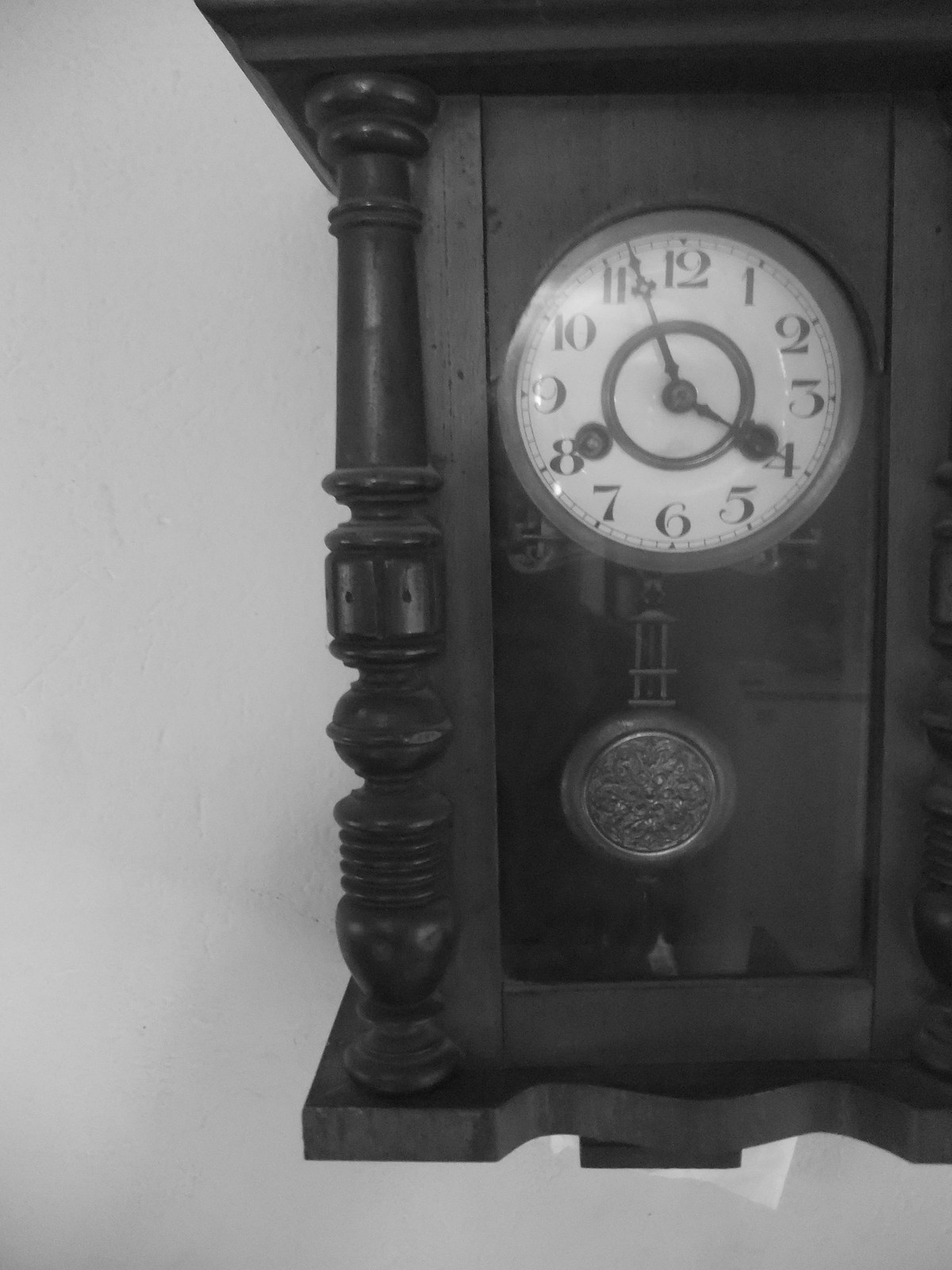This photograph showcases an antique grandfather clock, likely derived from Vienna or Germany, positioned against a white wall. The clock is predominantly black, possibly a dark mahogany wood, but it appears black in the image. The clock exhibits a refined structure with its prominent columns on both the left and right sides. The left column is fully visible, while only a portion of the right column can be seen. The clock's top is wide and angled, whereas the base is small and curves inward elegantly at the middle.

The main feature is a small, white clock face adorned with large black numerals from 1 to 12. The delicate, ornate hour and minute hands are crafted from metal. Notably, the time displayed is 4:57. The clock face also features metallic elements, including two round brass circles positioned above the four and eight, and another circular metal piece at the center.

A highlight of this clock is the pendulum, visible through a small glass encasement at the bottom. This pendulum, depicted as a large, round, hanging disc, is intricately detailed with ornate scrolling and imagery. The design elements evoke the charm and craftsmanship typical of traditional European timepieces.